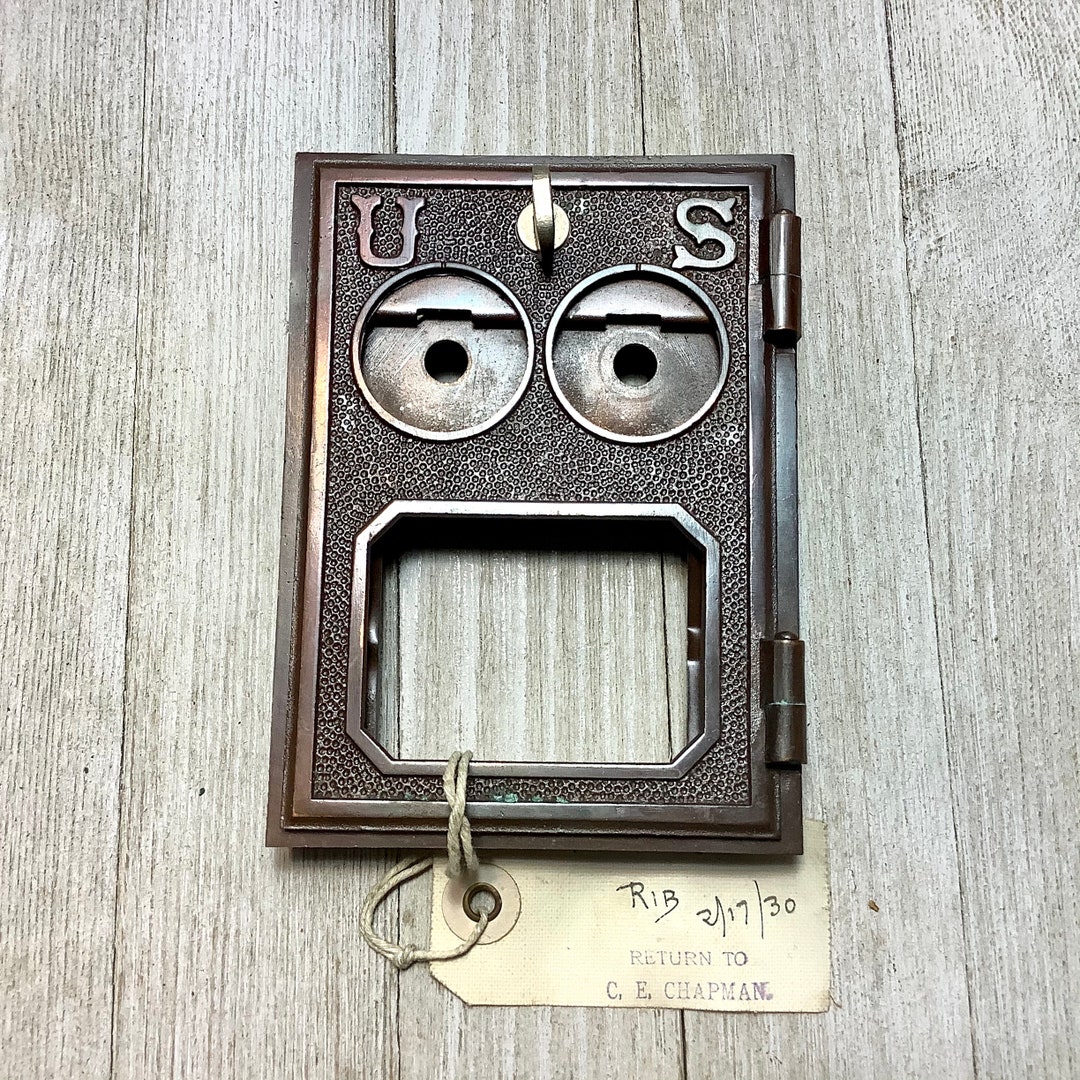This detailed photograph showcases a vintage brass door from an old U.S. mailbox, positioned on a weathered gray wooden table. The mailbox door, square in shape and crafted from a heavy, dark brown metallic material, is adorned with ornate embossed letters "U" and "S" at the top corners. Below these letters, two circular holes suggest places where dials or fixtures might have once been attached. The base of the door features a rectangular cutout, likely intended for a name plaque. Attached to the door is a soiled white string holding a white tag that reads, "R.I.B. 2-17-30. Return to C.E. Chapman." The overall setup, with the aged wood background and the meticulous details of the door, gives a rich, historical feel to the image.